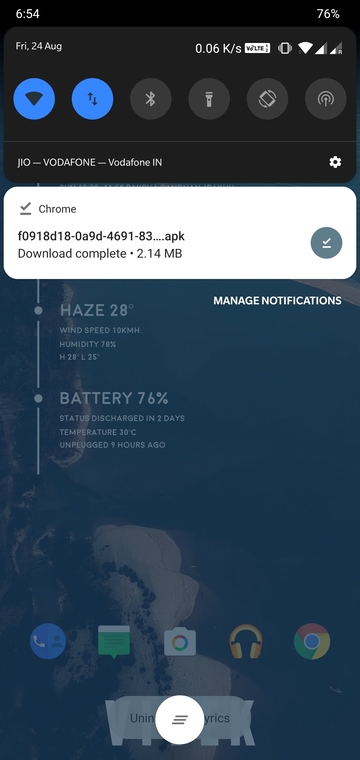**Descriptive Caption:**

This image is a screenshot of the notification section from a mobile phone. The interface features a black header with a row of small icons. Starting from the left, the first two icons have a blue background, indicating active functions, while the remaining icons, including a Bluetooth and a flashlight icon, have a gray background, denoting inactive states. The top section of the screen displays the date "Friday, 24th of August" on the top left, and on the top right, it shows icons for battery level, cellular signal, and Wi-Fi signal. 

Directly beneath the black header is a series of icons where the first few are blue, followed by icons with a gray background. Key notifications are displayed prominently in a white pop-up window, indicating that a "Chrome download is complete" with a file size of 2.14 megabytes. 

The phone's background wallpaper features a detailed aerial view of an island with varying shades of blue, creating a visually appealing theme. At the very top of the screen, weather information is shown, stating "Haze, 28°C" and the battery status is visible at "76%". Beneath the notification bubble, there is an option labeled "Manage Notifications."